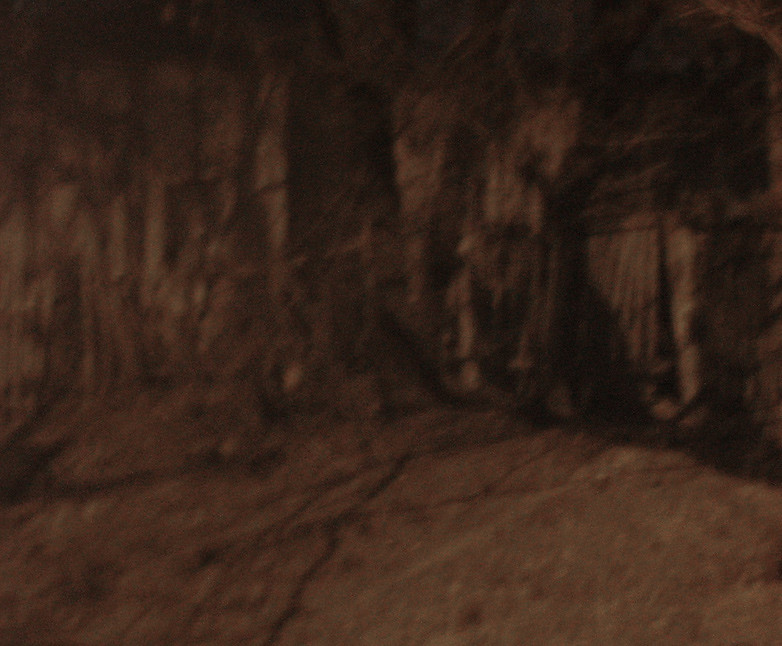In this nighttime photograph, the foreground features a section of gray concrete, noticeably pitted and marred with white spots, indicative of age and wear. The surface texture offers a stark contrast to the surrounding environment. In the background, densely packed overgrown branches and vines claw their way towards an indistinct wooden structure, hinting at nature reclaiming man-made spaces. The poor lighting and grainy quality of the image add an air of mystery, making it challenging to discern precise details of the scene. Nonetheless, the encroaching vegetation suggests a long-abandoned space being steadily overtaken by the natural world. The overall ambiance is one of eerie desolation, capturing a moment suspended in time.